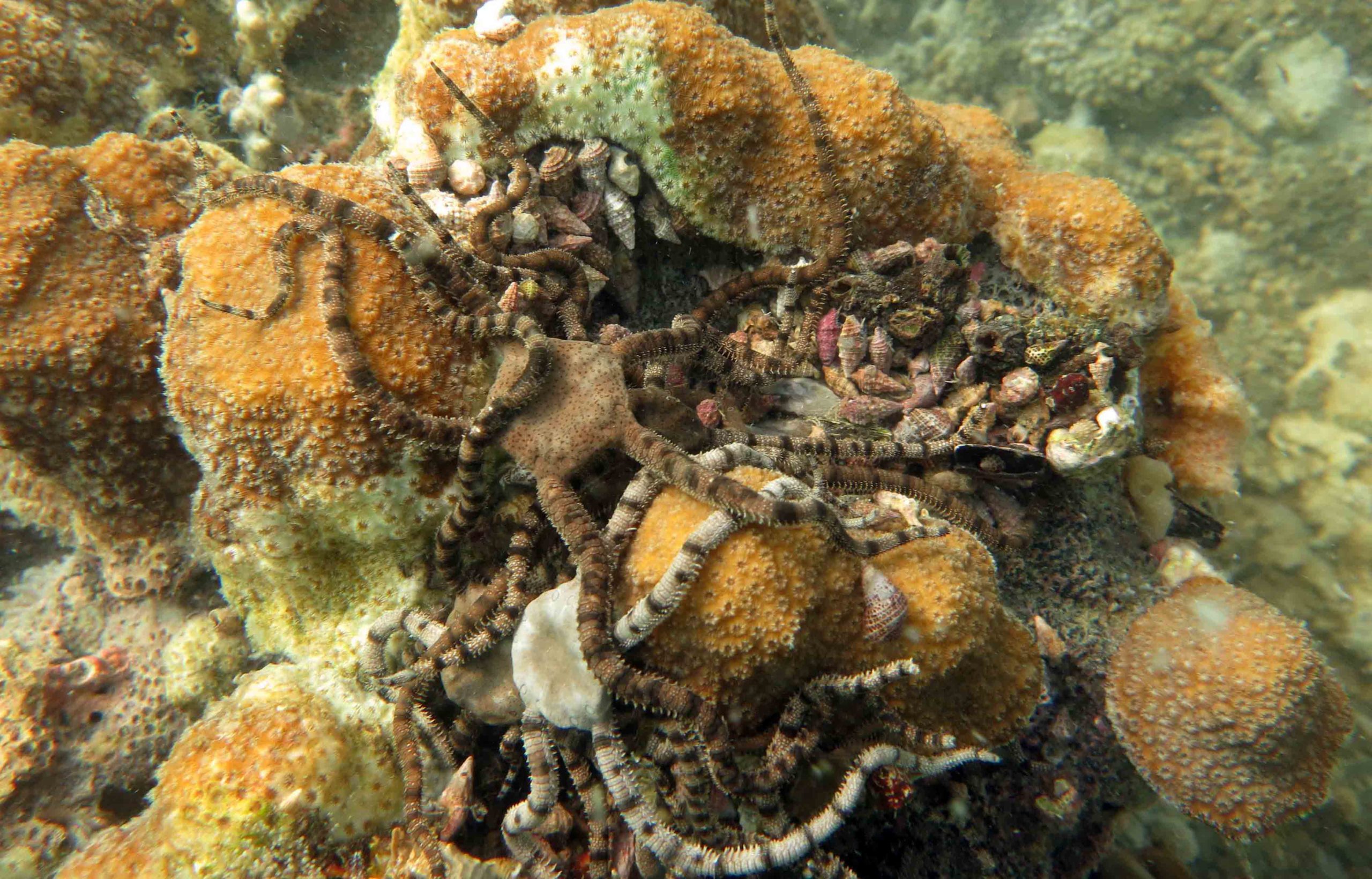This detailed underwater photograph showcases a vibrant scene at the ocean floor. Central to the image are two unique sea creatures, potentially small octopuses or squids, distinguished by their pentagonal-shaped bodies and multiple long tentacles, extending from each point of their bodies. The first creature is predominantly white with black splotches on its legs, while the second is a rich brown adorned with black splotches, rings, and circles on its tentacles. These creatures are nestled among a colorful coral formation, which is primarily orange with some white splotches. Scattered among the coral are numerous seashells, hinting at the biodiversity of the habitat. The coral appears to be bound to tan and light brown rocks, creating a textured and detailed backdrop. The clear water, with a slight greenish hue in deeper areas, provides a serene environment allowing for an unobstructed view of this vibrant underwater landscape.